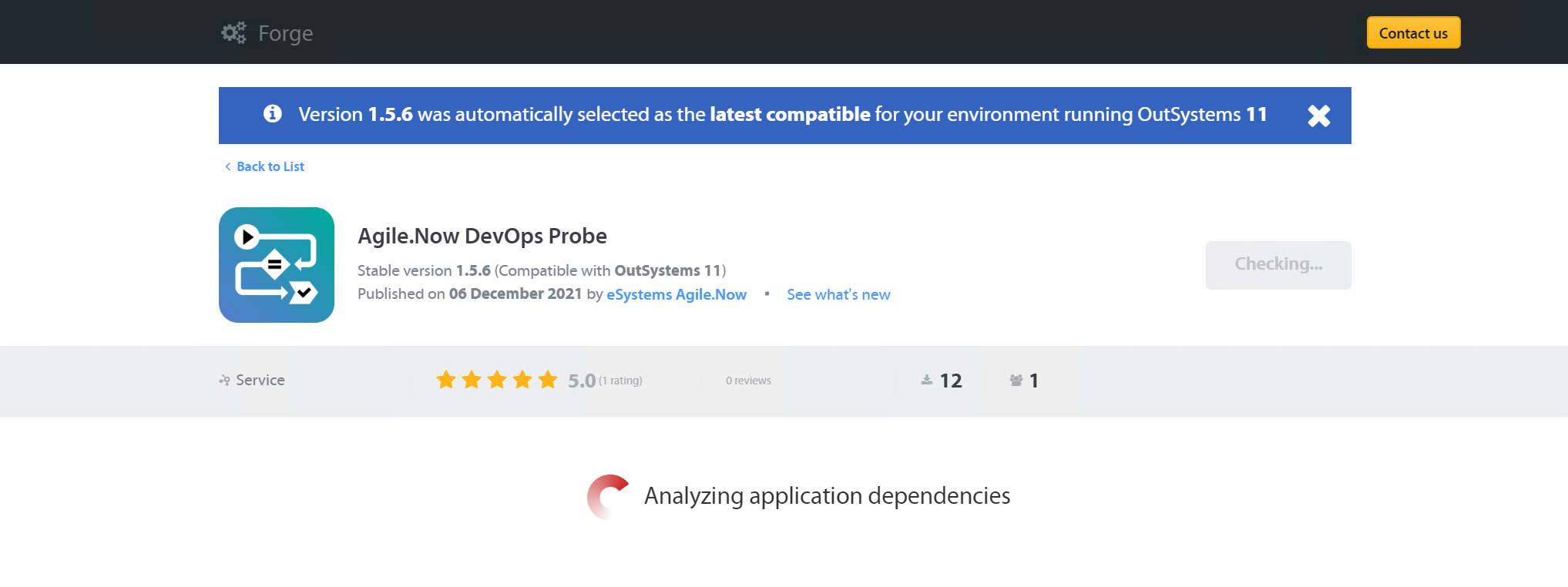Screenshot of a Website - Detailed Caption:

---

The screenshot represents a webpage featuring a dark-themed header with a black background. Prominently displayed on the header are three gears: one larger gear positioned on the left and two smaller gears stacked vertically to the right. Adjacent to these gears is the word "Forge" presented in a gray-colored font. To the far right of the header is a "Contact Us" option in black letters, immediately below which there is an orange-yellow button.

Beneath the header, there's a medium-blue horizontal rectangle bar that is narrower than the header. This bar contains an icon of an eye, colored in blue with a surrounding white circle. The bar displays the message: "Version 1.5.6 was automatically selected as the latest compatible for your environment running OutSystems 11," followed by an 'X' which possibly serves as a close button for this notification.

Below this notification bar is a navigation element, starting with a left-pointing arrow indicating "Back to list." The section underneath features an app icon decorated with various symbols: a triangle, an equal sign, a check mark, and assorted arrows—some within circles and diamonds, others doubled and pointing right.

Displayed next is content related to the application "Agile.now," indicating it is a DevOps probe tool. Specific details include:
- Stable version 1.5.6
- Compatibility with OutSystems 11
- Publication date: 06 December 2021
- Publisher: eSystems
- Further info link: "See what's new"

A gray bar beneath this information holds a symbol representing service quality, showcased by a 5-star rating—all stars are lit indicating a score of 5.0, based on one rating with zero reviews. There is also a download icon close by, resembling a small bar or a basket with a downward arrow. Adjacent, there's an icon depicting a box with various items appearing to emerge from it, tagged with the number 12.

Lastly, there is a spinning graphic that is depicted as slightly more than a half-circle, transitioning color gradients from dark red through light red to white, paired with the text "Analyzing application dependency."

---

This caption provides a meticulous breakdown of the webpage's visual and textual elements, ensuring a clear and comprehensive description.